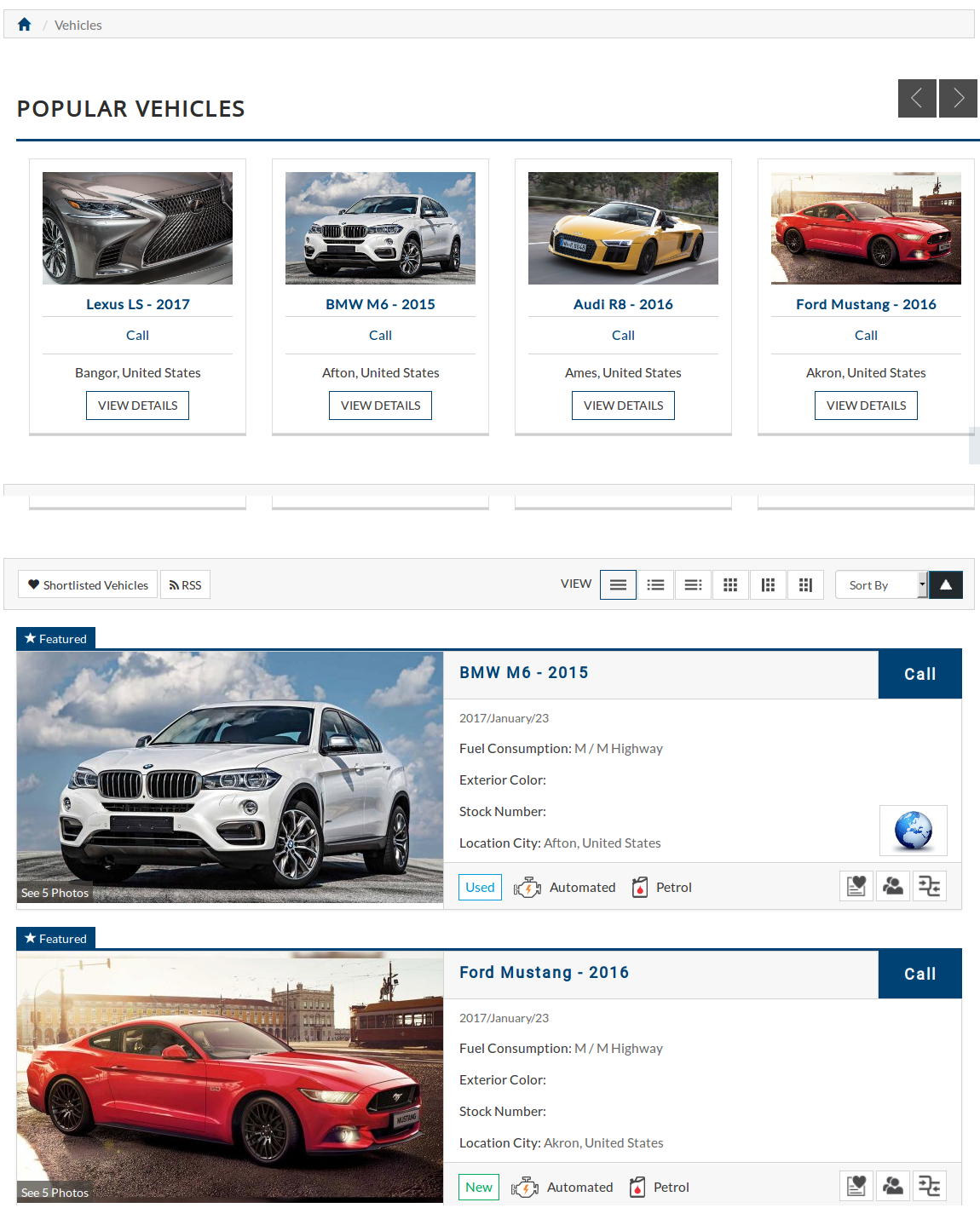The screenshot displays a website interface. In the upper-left corner, there is a "Vehicles" section adjacent to a "Home" button. Directly below this, the text "Popular Vehicles" is prominently displayed in black letters, with a blue horizontal line running from left to right underneath it.

Beneath this blue line, there are images of four cars arranged in a row from left to right, each accompanied by their respective names underneath. The cars featured are a gray 2017 Lexus LS, a white 2015 BMW M6 crossover, a yellow 2016 Audi R8 convertible, and a red 2016 Ford Mustang.

Below these images is an indication of another page labeled "Page 2." This section, titled "Shortlisted Vehicles," appears in the upper-left corner next to a heart icon. To the right of this title, differing view options are available, displaying cars in left, centered, and right-aligned formats. In the upper-right corner, there is a sorting field to organize the vehicles.

Listed below in a vertical sequence are the previously mentioned white 2015 BMW M6 and the red 2016 Ford Mustang, displayed one above the other.